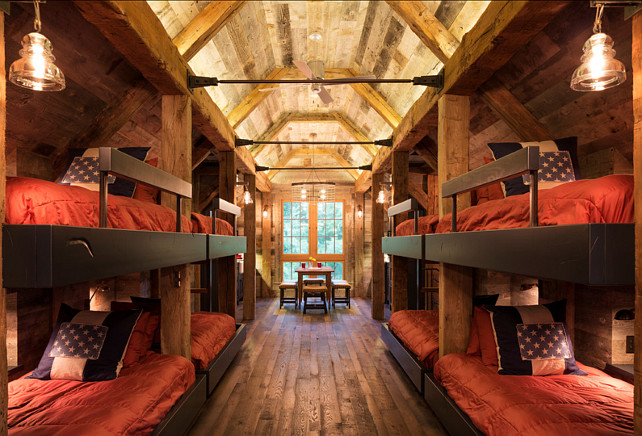This color photograph captures the interior of a bunkhouse with a slightly arched high ceiling made of light brown wood planks, supported by large wooden beams. The darker brown wooden floor complements the ceiling's rustic charm. Lining both sides of the narrow cabin aisle are built-in bunk beds, extending back as far as the eye can see. The bunk beds, crafted from dark wood and almost black in color, feature individual light fixtures above each one. Each bunk exudes coziness, adorned with wrinkly reddish-orange bedspreads and pillows decorated with white polka dots on a blue background. The top bunk beds come equipped with black safety rails and wood stops to prevent rolling out. In the far distance, a table with benches sits against a backdrop of wide, tall windows, bringing natural light into the cabin. The overall atmosphere is one of warm, communal living in a snug, wood-framed structure.